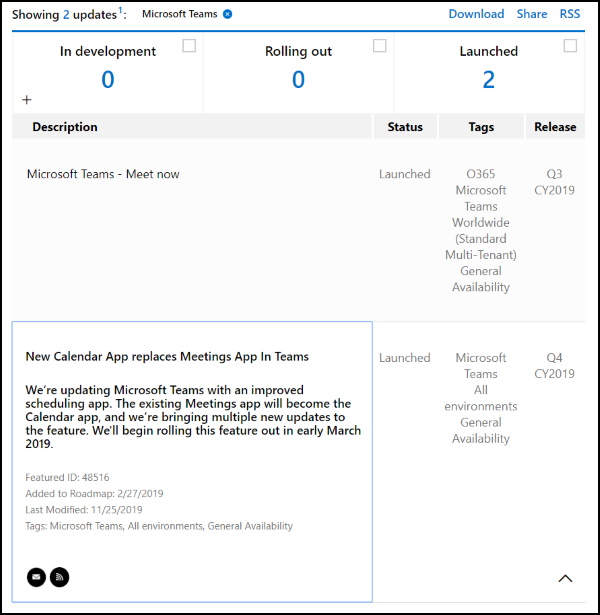Screenshot from Microsoft Teams Release Notes:

![Image Description]
A square-shaped screenshot with a thin black border displays a Microsoft Teams information page. The background is primarily white, with a cobalt-blue horizontal line near the top. Above the blue line, the page reads "Showing two updates," where the number "2" is in blue, and the rest of the text is in black, followed by a superscript "1", likely indicating a footnote elsewhere on the page. 

Below this, the Microsoft Teams logo and name appear, followed by ample white space. There are three blue hyperlinks: "Download," "Share," and "RSS."

Beneath the blue line, there are three headers with accompanying gray boxes that seem selectable but are currently not checked. The headers are:
1. "In Development" with a blue "0"
2. "Rolling Out" with a blue "0"
3. "Launched" with a blue "2"

Following this is a light gray bar segmented into four sections labeled: "Description," "Status," "Tags," and "Release." The "Description" section is the largest, spanning most of the bar's length. 

Details under this bar include:
- **Description:** Microsoft Teams - Meet Now
- **Status:** Launched
- **Tags:** O365, Microsoft Teams, Worldwide (Standard Multi-Tenant), General Availability
- **Release:** Q3 CY 2019

The bottom half of the page features a light blue-outlined rectangle with the following update:
- **Title:** New Calendar App Replaces Meetings App in Teams
- **Content:** We are updating Microsoft Teams with an improved scheduling app. The existing Meetings app will become a Calendar app, and multiple new updates will be added to this feature. We will begin the rollout in early March 2019.

Beneath this descriptive content in small font, there is metadata:
- **Feature ID:** 48516
- **Added to Roadmap:** 02.27.2019
- **Last Modified:** 11.25.2019
- **Tags:** Microsoft Teams, All Environments, General Availability

Additionally, two black circular buttons are in the bottom-left corner, one with an envelope icon (likely for email), and the other with an unclear icon. On the bottom-right, corresponding details for the new Calendar app mention:
- **Status:** Launched
- **Tags:** Microsoft Teams, All Environments, General Availability
- **Release:** Q4 CY 2019